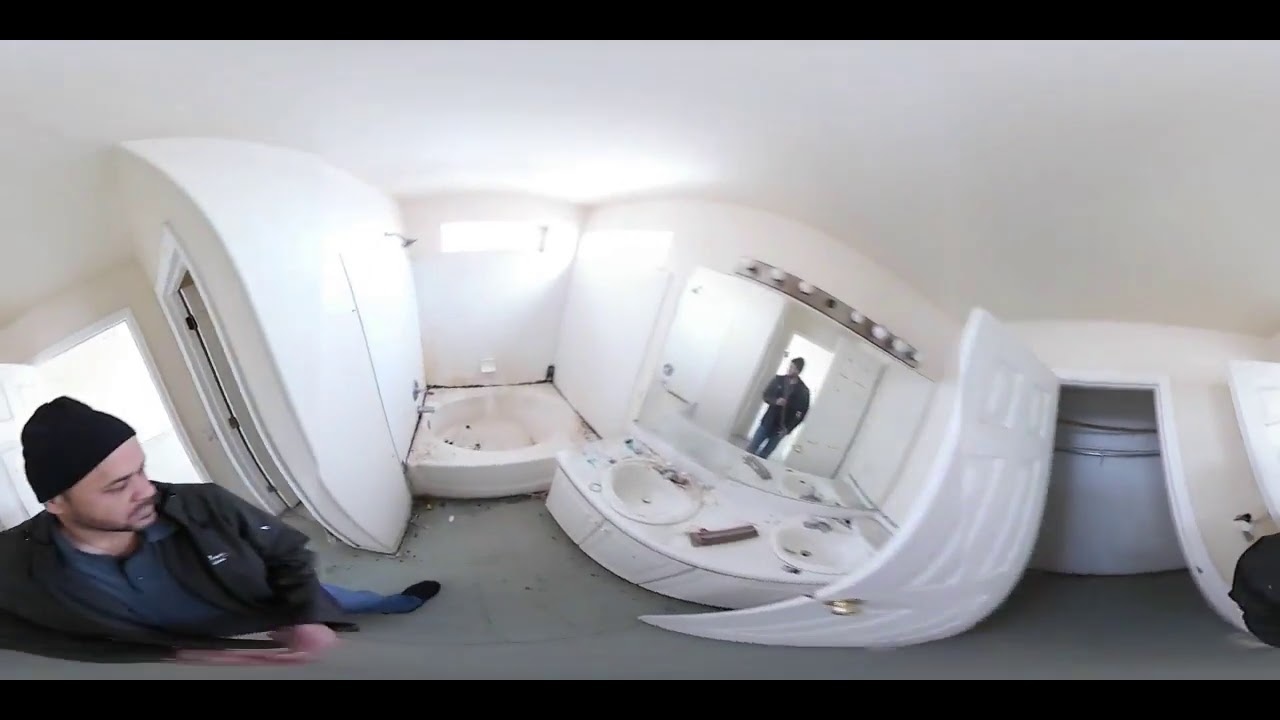This is a horizontal-rectangular image showcasing a somewhat unconventional-shaped white room with curved walls, which might suggest the use of an unusual lens or an architecturally atypical structure. Prominently featured in the lower left corner is a man dressed in black attire, including a black hat, jacket, and shoes. He has a mustache and a closely shaven beard, and his reflection is visible in a bathroom mirror located towards the right of the image. 

The room appears to be a bathroom, featuring two white sinks with an ambiguous object between them, a cluttered bathtub to the left, and some debris scattered on the floor, suggesting a state of disrepair or ongoing renovation. The bathroom elements, such as the sinks, cabinets, and vanity light above the sinks, all adhere to an all-white color scheme, enhancing the room's overall starkness. In addition to these details, there are multiple doorways visible, including one that leads to what resembles a closet on the right side of the image.

Overall, the scene combines elements of disarray with the detailed depiction of the man and his mirrored reflection, capturing the room’s intricate layout and unique aesthetic.